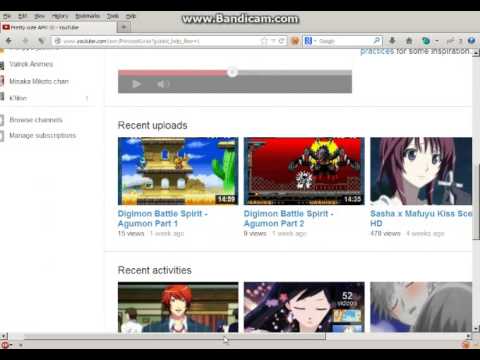The image showcases a webpage of the site www.bandicam.com. Due to the compact size of the image, the text is largely unreadable, and certain portions appear deliberately blurred. The top section prominently displays the Bandicam website's URL. Below the address bar, there's a search bar with text that is difficult to decipher.

Central to the image is a darker gray bar that seems to indicate media playback, evidenced by a red progress bar that's about halfway filled. Directly beneath this bar is a section titled "Recent Uploads," featuring various cartoon characters, including figures from the series "Digimon" and "Battle Spirits," as well as characters identified as Sasha and Mayuka.

Following the "Recent Uploads" section is another segment labeled "Recent Activities," displaying additional cartoon figures. The characters in this section include a man with red hair, a girl with black hair, and two individuals with gray hair. On the left side of the image are multiple listings accompanied by small images, the details of which are not discernible due to the resolution.

At the bottom of the page, there's another gray bar. Within it, an arrow directs attention to the starting image in the "Recent Activities" row. The image concludes with a solid black bar at the very bottom, completing the website's interface depiction.